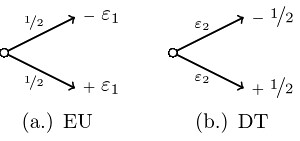This landscape-oriented image features a white background and presents an illustration resembling a mathematical or algebraic concept. 

On the left side, there is a circle with a vertical line extending upwards, ending in an arrow, and another vertical line extending downwards, also ending in an arrow. Above the upper arrow, the label reads "1/2" and "−e1", while the lower arrow is labeled "1/2" and "+e1". Underneath this diagram, there is the text "(A) EU" in capitals.

On the right side, an identical circle with vertical arrows is depicted. However, the labels differ; the upper arrow is marked "e2" and "−1/2", and the lower arrow is labeled "e2" and "+1/2". Below this right-side diagram, the text reads "(B) DT" in capitals.

This detailed illustration conveys variations of a mathematical concept with precise annotations and symmetric visual elements, likely highlighting differences in algebraic equations or transformations.